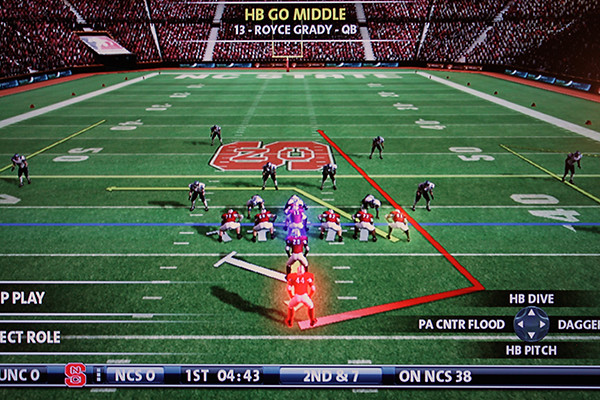This color screenshot from an unknown football-themed video game captures an intense moment on the field. At the center stands a player, glowing red to indicate their importance or current selection. Surrounding him are several teammates poised in a crouched stance, wearing red jerseys and white pants, preparing for the next play. The opposing team, although not clearly visible, is discernible in dark uniforms. The backdrop features a stadium packed with spectators, adding to the atmosphere of a significant game.

At the top of the screen, game details are provided: "HB Go Middle 13 Royce Grady QB." The bottom of the image is filled with various icons and game information. The score is displayed as "NCS 0," and it notes the current status, "1st 04:43 2nd and 7 on NCS 38." Additionally, there is a directional icon with four arrows, each labeled with different play options: "HB Dive" for the top arrow, "PA Center Flood" for the left, "HB Pitch" for the bottom, and "Dagger" for the right. This screenshot vividly encapsulates a strategic moment in the game, showcasing both teams ready for action amidst a dynamic stadium backdrop.